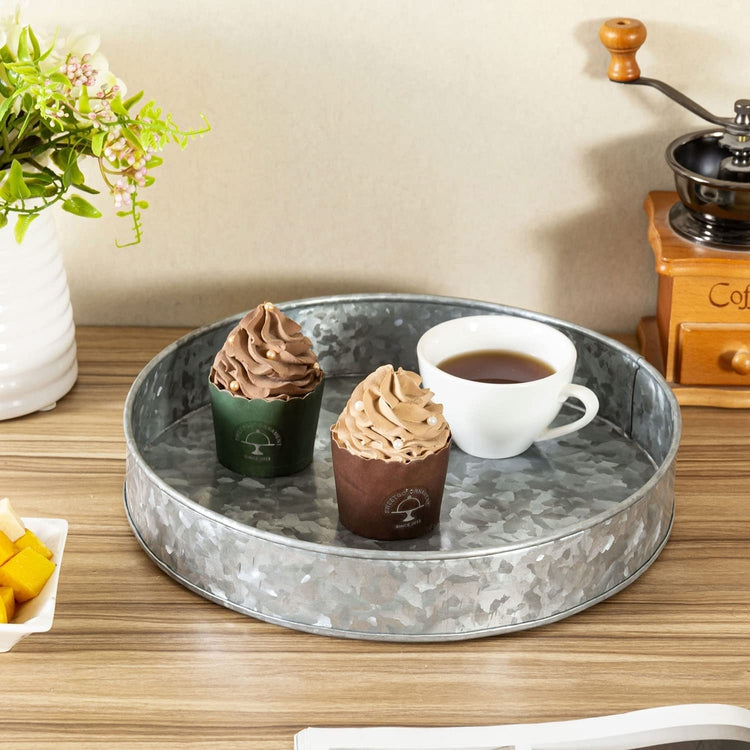This photograph captures a cozy domestic snack setup featuring a galvanized metal serving tray with a slightly raised rim, adorned with a delicate gray floral pattern. Central to the tray is a short white mug of coffee or tea, characterized by a wide, round opening that tapers slightly towards the base. Alongside the mug are two cupcakes, each topped with mocha frosting—one with a slightly darker hue than the other. One cupcake is wrapped in a hunter green cupcake paper, while the other is housed in a chocolate brown wrapper bearing a bakery logo.

The tray rests on a simple brown wooden table. Behind the tray, a vase with pink flowers and green leaves adds a touch of freshness, and beside it sits a dish filled with cubed pieces of bright yellow fruit, possibly mango or peaches. To the right, partially cut off, there is an old-style wooden coffee grinder with a metal container and a wooden handle. The background wall is a light beige, complementing the earthy tones of the setup. Additionally, the bottom right corner of the image reveals the edge of an open magazine or book, adding a homely touch to this inviting scene.